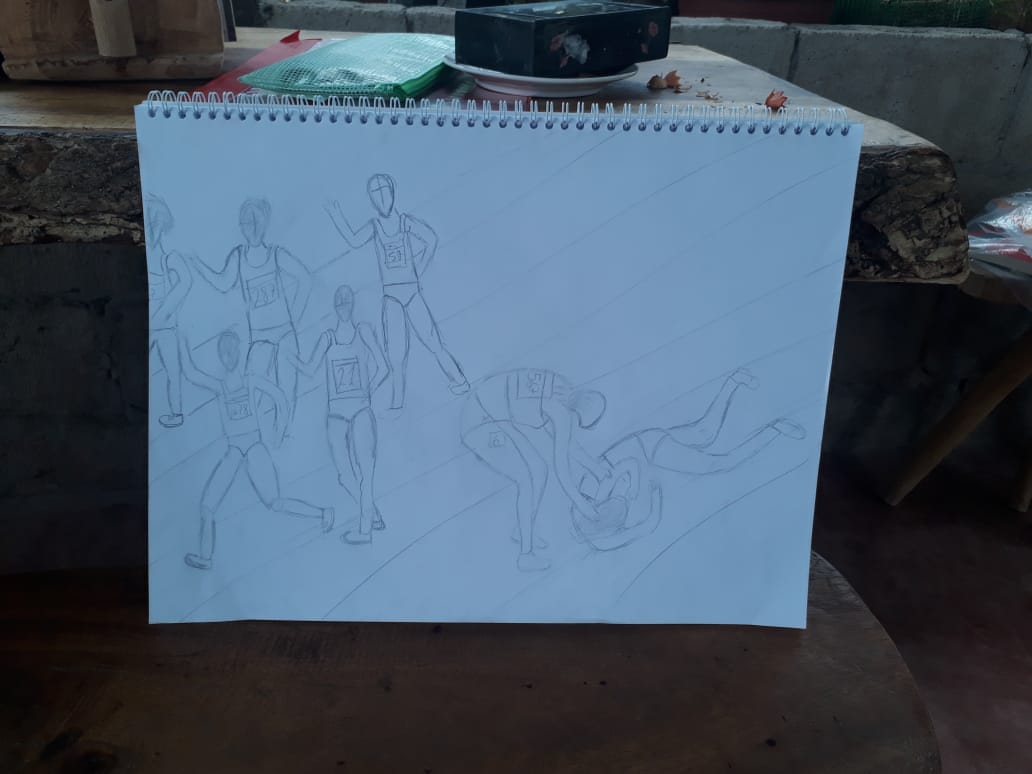The image depicts a detailed pencil sketch on a white, wire-bound sketchbook, propped horizontally against a rough stone tabletop, possibly leaning on a chair or bench. The sketch captures a scene from a running race on a six-lane track. Five runners are depicted actively running towards the left side of the page, although some appear to be standing due to the drawing's rough lines. Their attire includes sleeveless shirts and running shorts, each with a square number—one visible number being 27—on their chests. On the right side, a pivotal moment is illustrated: one runner has fallen to the ground, while another is bent over, assisting them. The background includes a green pencil case, a white plate with a black box on it, and pencil shavings scattered across the stone plinth. The sketch lacks facial details, adding a raw, unfinished aesthetic to this moment of sportsmanship captured in mid-race.